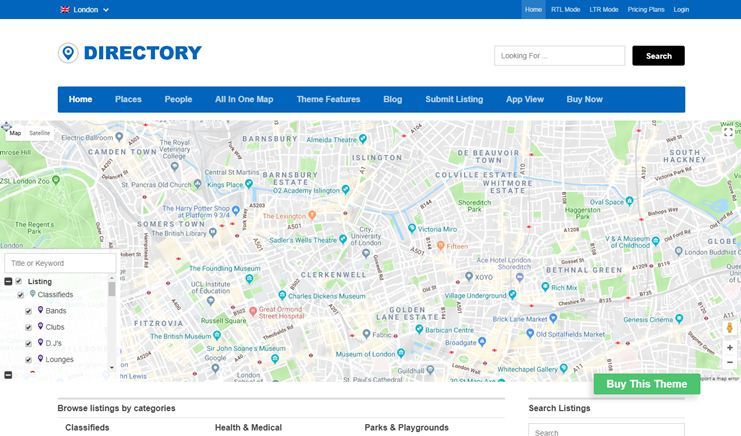Screen capture of a map interface showcasing various features and navigation options. At the top-left corner of the ribbon, the heading "London" is visible, indicating the city being displayed. To the right, the ribbon includes several navigational buttons labeled: Home, RTL Mode, LTR Mode, Pricing, Plans, and Login.

In the main field below, the left side features the label "Directory," followed by a search window with a search button and a black rectangle adjacent to it. A secondary ribbon with multiple tabs is positioned below this, including options such as Home, Places, People, All in One Map, Theme, Features, Blog, Submit Listing, App View, Buy Now, with the Home tab currently selected.

The central portion of the screen displays a highly detailed street map, presumed to be of London. On the lower-left side of the map, a pop-up window titled "Listings" presents several checked categories: Classified, Bands, Clubs, DJs, London. 

In the lower-right corner, there is a prominent green button labeled "Buy This Theme." The map appears to be an interface potentially for a website, offering navigation and category-browsing functionality.

At the very bottom, the heading "Browse Listings by Category" is visible, followed by three tabs labeled: Classified, Health and Medical, and Parks and Playgrounds.